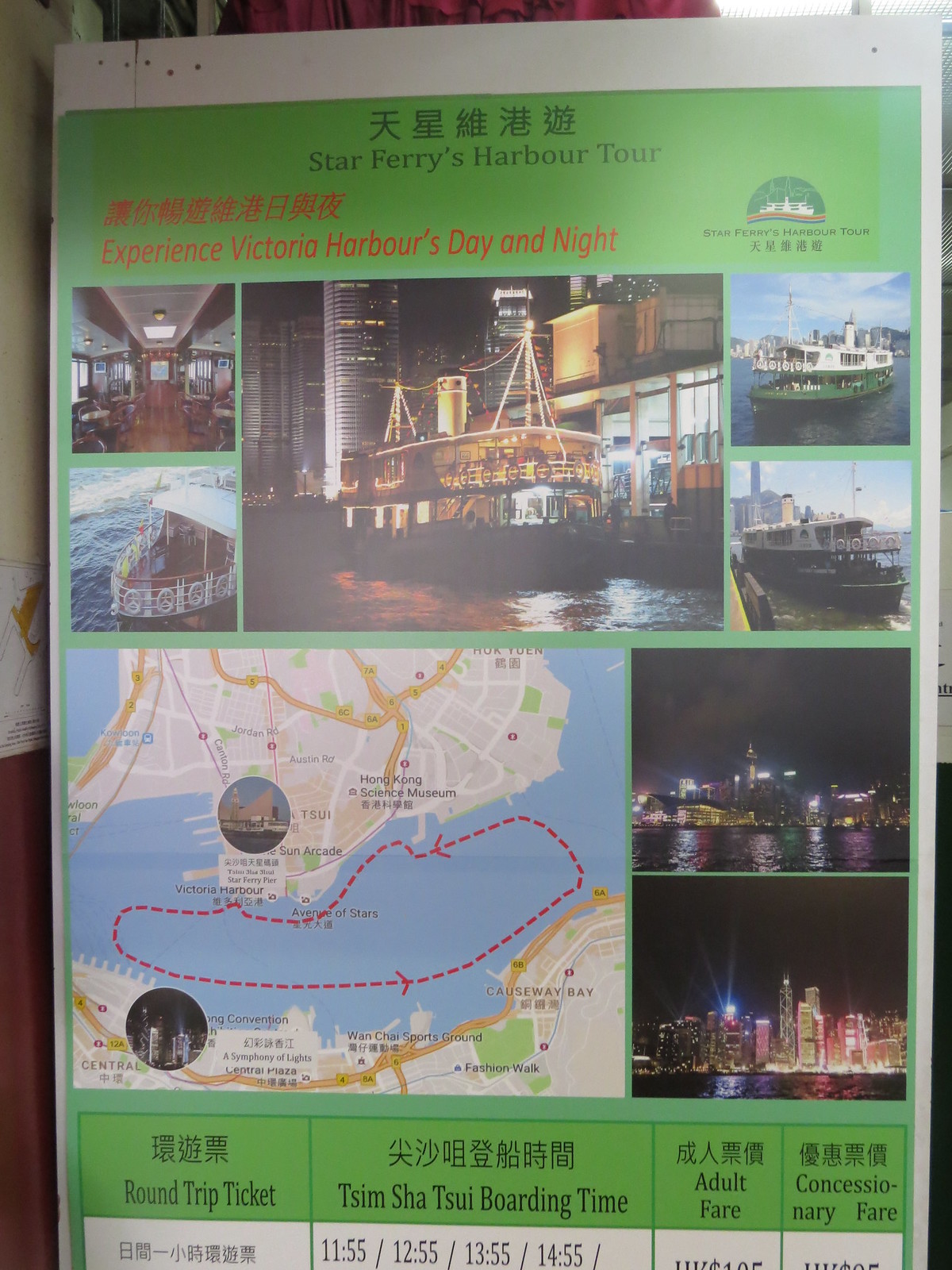The photograph depicts a poster prominently displayed at a pier or ferry stop, likely a tourist destination in Asia, as suggested by the presence of Chinese characters. The poster has a white border and a green background. At the top, Chinese characters are followed by an English title that reads "Star Ferries Harbor Tour." Beneath this, a subtitle in red text states "Experience Victoria's Harbors Day and Night." The poster features a montage of images showcasing the ferry's interior and exterior, as well as views of the harbor during both day and night. A logo that reads "Star Ferries Harbor Tour" is located on the right side. Towards the bottom left of the montage, there is a map showing a circular route marked by a red dotted line, indicating the ferry's path between two landmasses separated by water. Below the images and map, a table provides detailed information on round-trip ticket prices, boarding times at Tsim Sha Tsui, adult fares, and concessionary fares. The map likely depicts Hong Kong's Victoria Harbor, further emphasizing the poster's role as a guide for tourists exploring the harbor's scenic views.